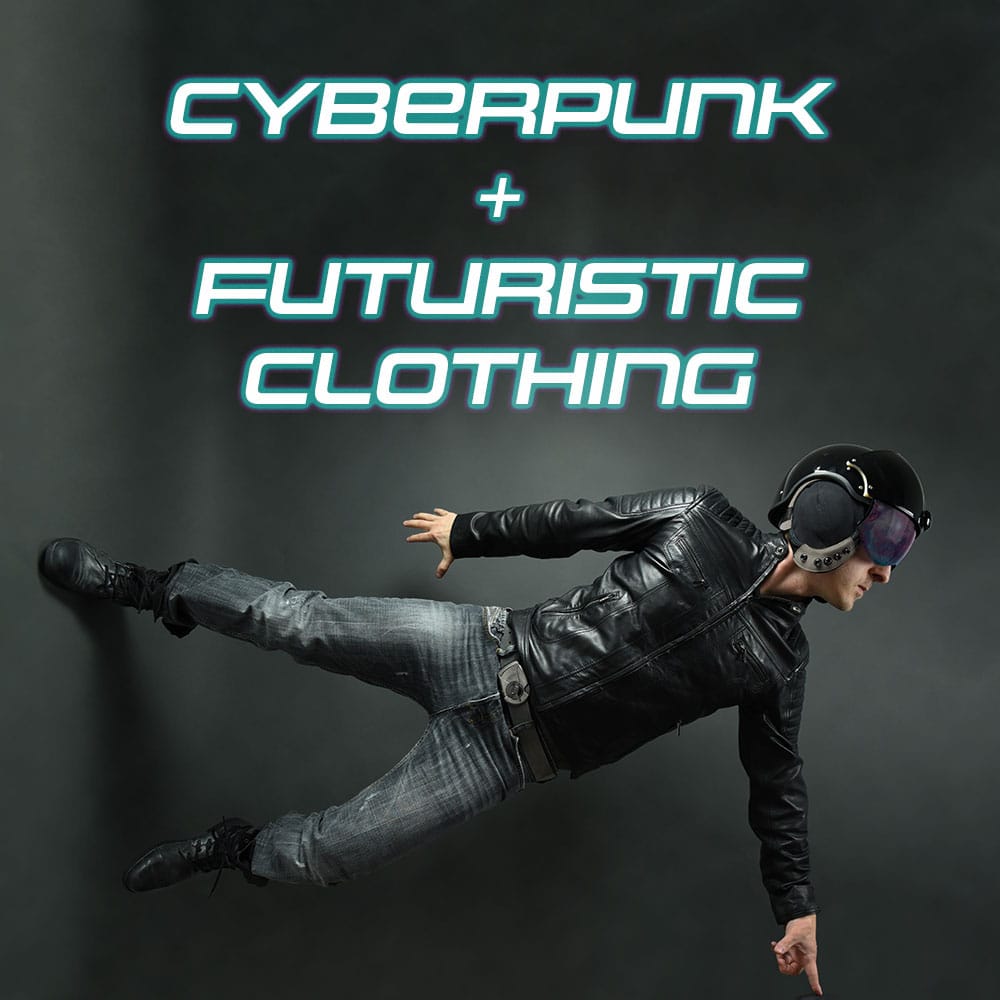The advertising poster features a dark gray background with the text "Cyberpunk + Futuristic Clothing" displayed prominently in a futuristic, white font outlined in green, occupying the upper half of the image. Dominating the lower half is an intriguing visual of a man oriented horizontally, as if defying gravity. Positioned with his feet on the left side and head towards the right, the man is clad in a black leather jacket, blue jeans, and black boots. His black helmet, fitted with purple goggles, enhances the cyberpunk aesthetic. His left hand points downward, while his right hand reaches slightly back, palm facing the wall behind him. A distinguishing feature includes a grayish, chrome-colored belt buckle visible just below his snug jacket. The man’s pose and attire, combined with the overall design, vividly evoke a futuristic and rebellious cyberpunk theme.